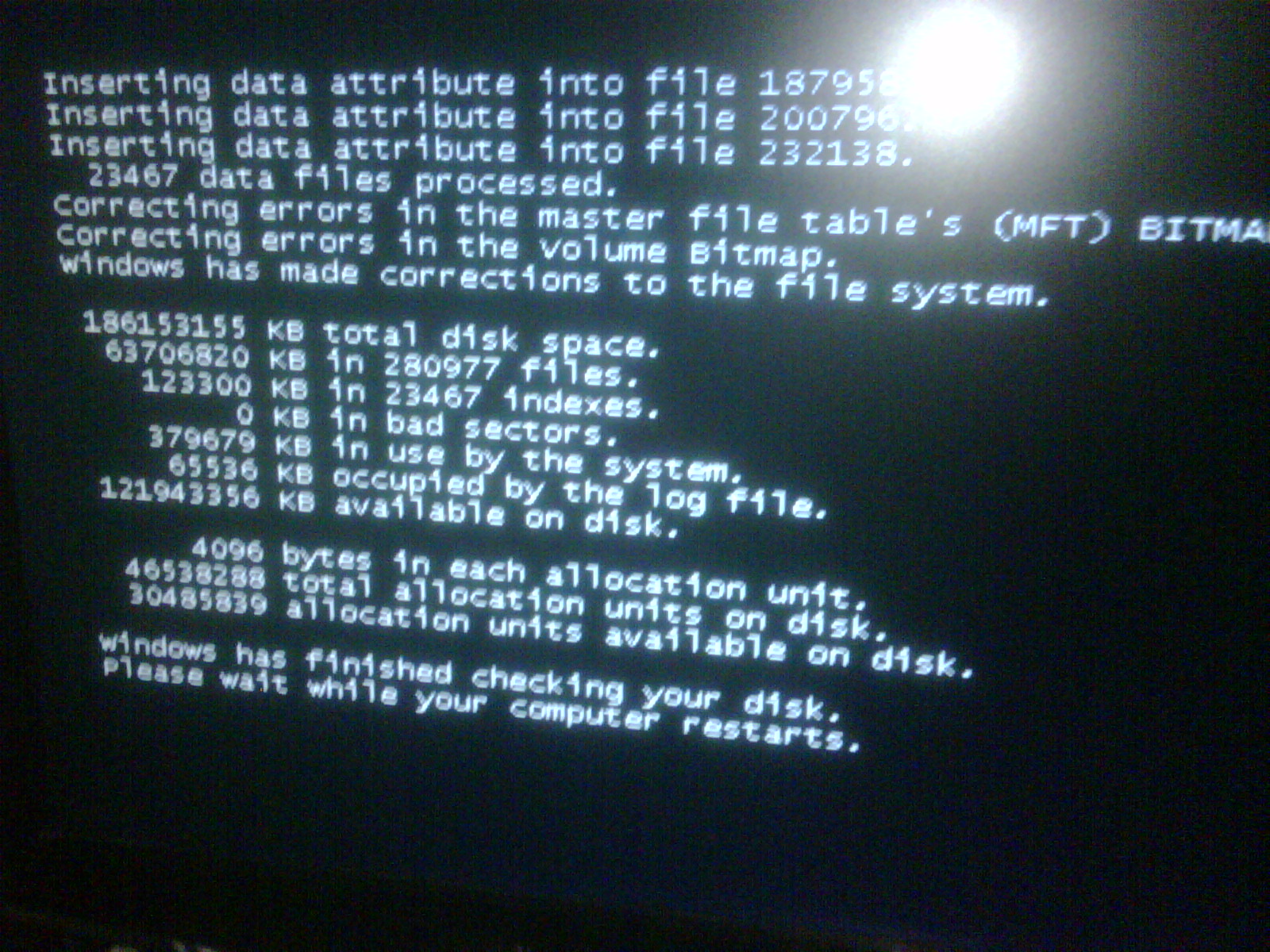The image is a close-up photo of a computer screen, displaying a typical black background with numerous lines of white text, likely from a disk check or system error correction process. Prominently, it features messages such as "Inserting data attribute info file 187958", "Inserting data attribute info file 2007967", and "Inserting data attribute info file 232138." Following these, it states "23,467 data files processed" and "Correcting errors in the master file table (MFT bitmap)", along with "Correcting errors in the volume bitmap." Subsequent lines show system corrections: "Windows has made corrections to the file system," with detailed storage data like "186,153,155 KB total disk space," "63,706,820 KB in 280,977 files," "123,300 KB in 23,467 indexes," "0 KB in bad sectors," "379,679 KB in use by the system," and "65,536 KB occupied by the log file." Other specifications include "121,943,356 KB available on disk," "4096 bytes in each allocation unit," and a summary of allocation units with "46,538,288 total allocation units on disk" and "30,485,839 allocation units available on disk." The concluding message reads, "Windows has finished checking your disk. Please wait while your computer restarts."